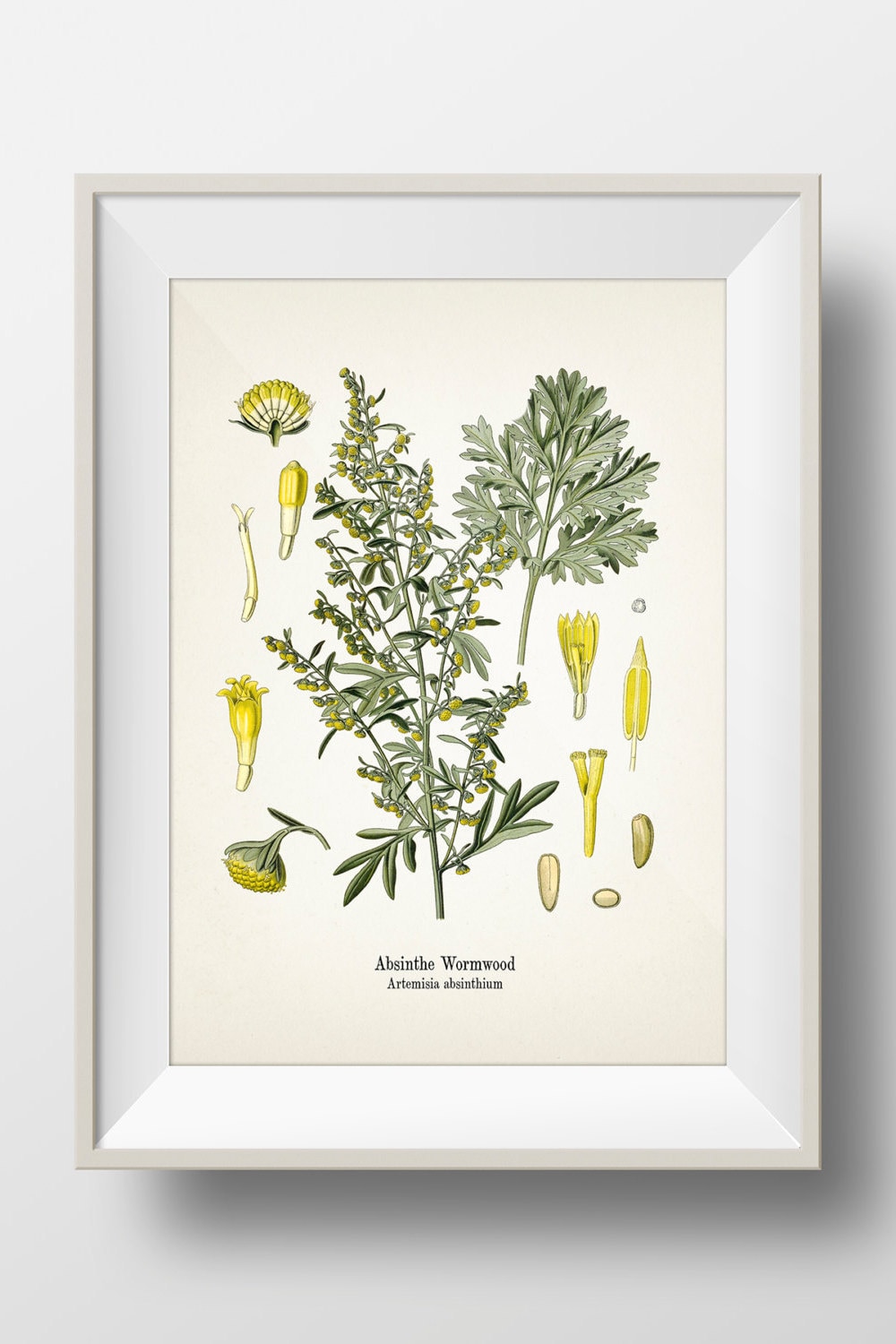This is a photograph of a framed botanical illustration of absinthe wormwood (Artemisia absinthium) on a white wall. The slightly off-white frame angles inward towards an ivory-colored canvas. The central drawing showcases a detailed depiction of the full plant, highlighting its yellow flowers and intricate leaves. Surrounding the main illustration are several smaller drawings representing various stages of the plant's development. On the left, individual yellow flowers progress from full bloom to unopened buds. To the right, there are detailed images depicting the plant's growth from seed to flowering. The bottom of the illustration features black text with the common name "Absinthe Wormwood" and the scientific name "Artemisia absinthium" in slightly smaller font. The entire composition, illuminated by a subtle shadow cast lower and to the right, conveys the intricate botanical details of this noteworthy plant.